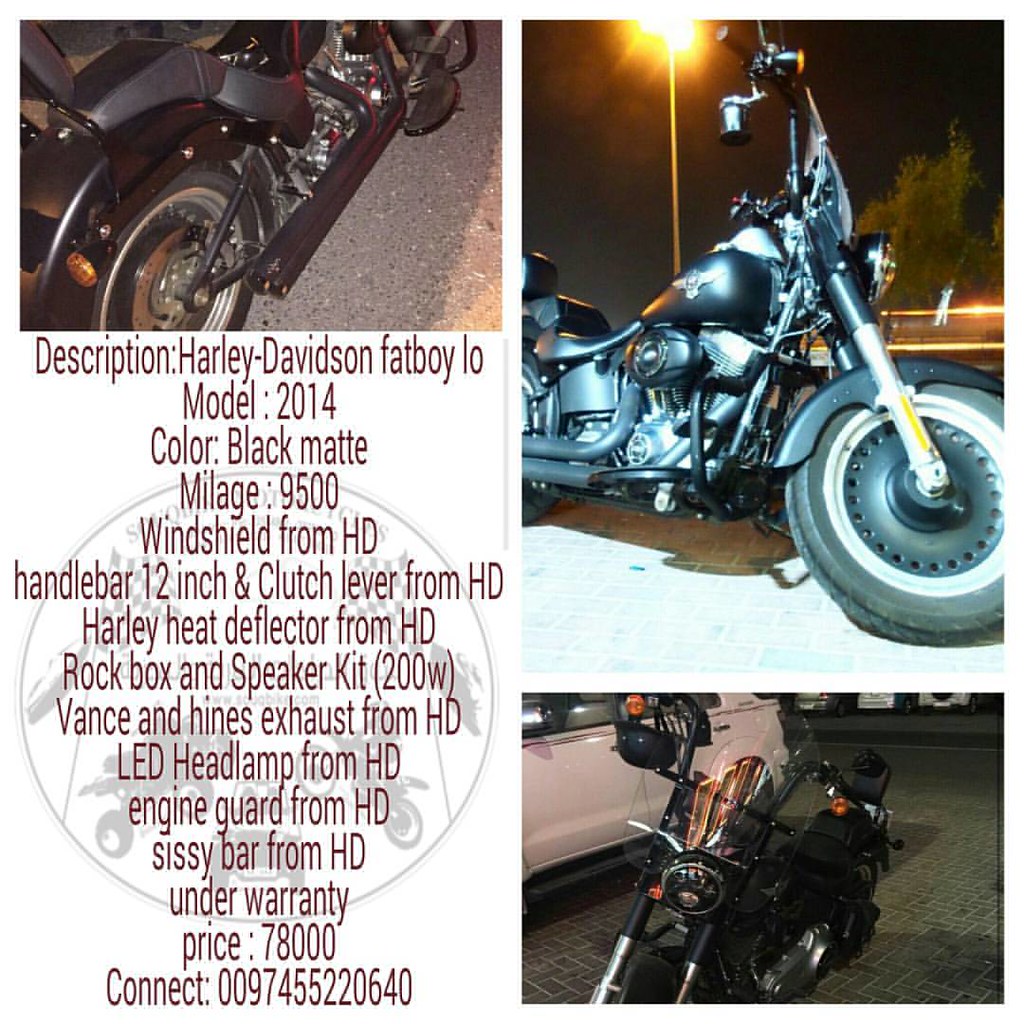A full-color print advertisement showcases three photographs of a Harley-Davidson Fat Boy Low motorcycle, model year 2014. All images feature dark-colored bikes, with the upper left photo showing only a partial view. The larger image on the upper right displays a striking metallic blue motorcycle, while the bottom right photo shows a dark motorcycle. The left side of the ad is filled with a detailed description: "Harley-Davidson Fat Boy Low, Model 2014, Color Black Matte, Mileage 9,500. Featured accessories include a windshield, 12-inch handlebar, clutch lever, heat deflector, rock box, 200-watt speaker kit, Vance and Hines exhaust, LED headlamp, engine guard, and sissy bar, all custom components from Harley-Davidson. It’s under warranty and priced at $78,000." A European contact number "00975422640" is provided for inquiries.